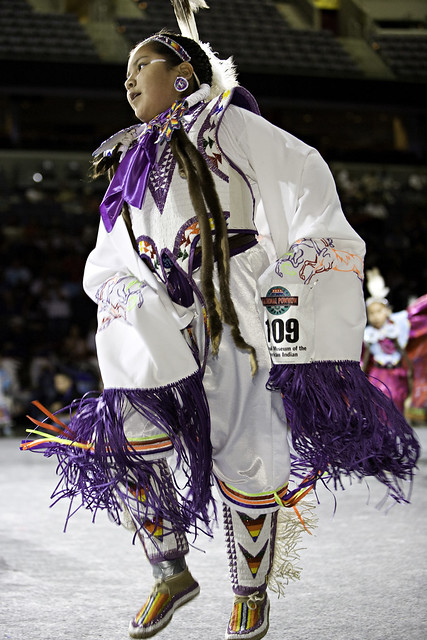In this vibrant image, a young Native American girl is captured mid-dance, gracefully facing the left with her mouth slightly open. Her striking black hair flows down to her hips, adorned with black and white feathers. She wears a white earring trimmed with purple, and a single white line is painted from the corner of her eye to her hairline. Her traditional attire is a voluminous, predominantly white garment reminiscent of an oversized gi, embellished with vivid, multi-colored designs. The sleeves of her outfit feature the number 109, identifying her as a competitor, and are accented with long purple tassels like those on pom-poms. Around her neck, she sports a purple satin bow or kerchief. Her feet are clad in moccasin-like boots, decorated with intricate native drawings in neon hues of yellow, orange, blue, and purple, creating a V-design on the shins and stripes on the toes. The backdrop reveals a blurred audience, along with another performer in pink. The girl appears to be participating in a traditional dance competition within an arena, performing on a textured white surface.